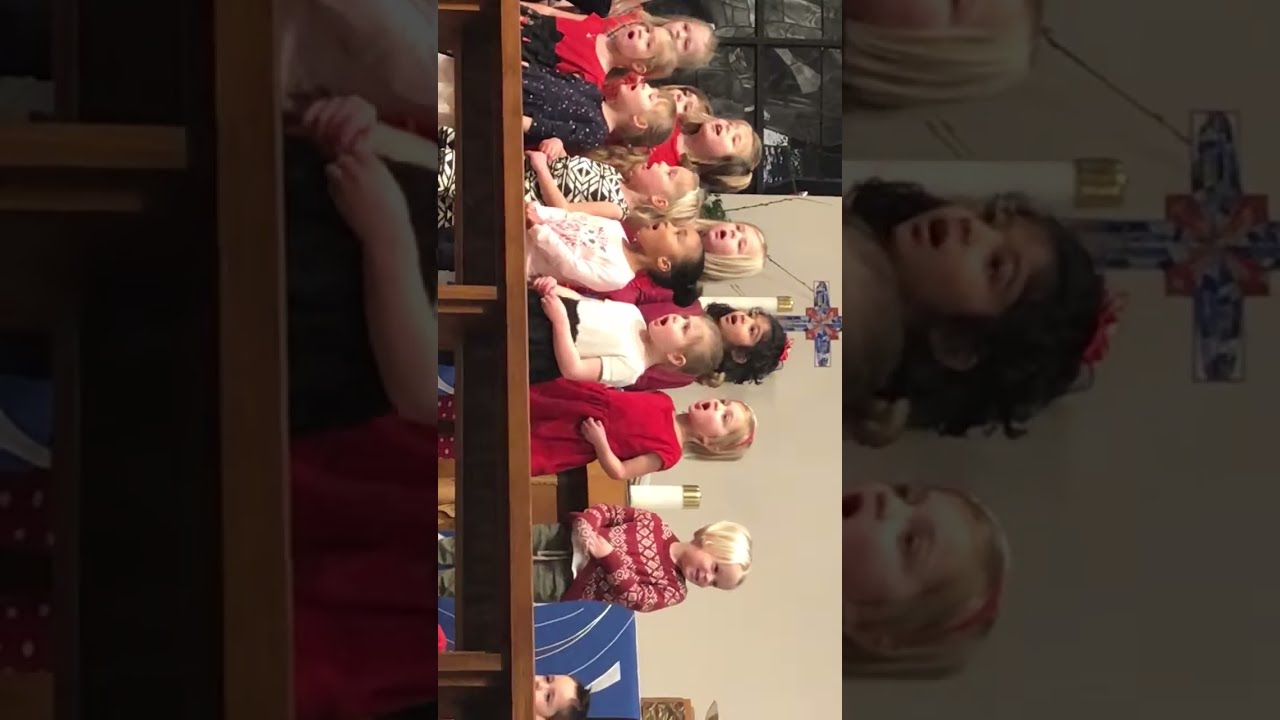The photograph, mistakenly taken or viewed sideways, displays a lively scene of young children, approximately two years old, gathered in a church setting. This detailed tableau features 12 children standing in a row in what appears to be a choir pew. The children, likely involved in a singing activity, are dressed in an array of fancy party dresses, with colors ranging from red, white, and black to a combination of these hues. In the background, a multicolored cross made of painted glass is prominently displayed against a white wall. Additionally, a podium with two lit candles is visible, contributing to the ambiance. Varied hair colors, from white blonde to dark brown, add to the visual diversity of the children. The photo captures not only the harmonious and festive spirit of the occasion but also the candid charm of its youthful participants.